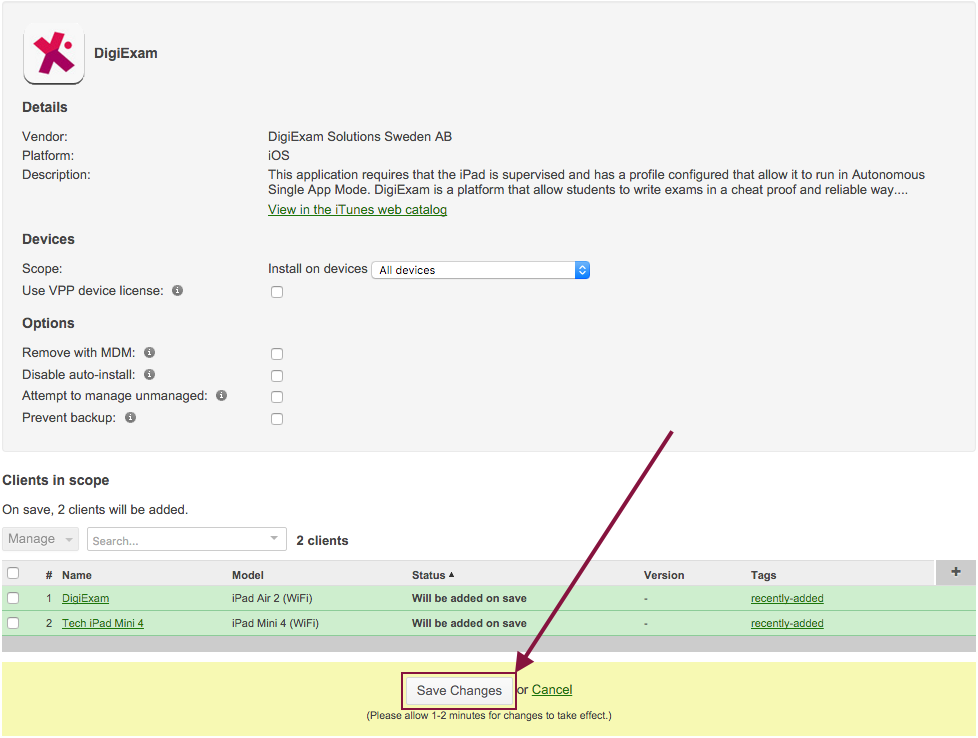This is a screen capture of a web page for the DigiExam platform. 

In the upper left corner, the heading "DigiExam" is displayed in black text. To the left of this heading, there is a white box with a gray border. Inside this box is a red "X" tilted at a five-degree angle, accompanied by a small red dot. The "X" features a light red color on the top half and a dark red color on the bottom half.

Below this area, there is a menu with various options:
- "Details Vendor Platform Description"
- "Devices Scope Use VPP Device License," accompanied by an information icon
- Options listed below:
  - "Remove" (with an MDM information icon)
  - "Disable Auto Install" (with an information icon)
  - "Attempt to Manage Unmanaged" (with an information icon)
  - "Prevent Backup" (with an information icon)

To the right of the menu, the content describes the DigiExam solution suite, aligned with ABIOS. This section informs users that the application requires the iPad to be supervised and equipped with a profile that allows it to operate in autonomous single app mode. DigiExam is introduced as a platform facilitating students to take exams in an efficient, cost-effective, and reliable manner.

Following this description, there is a green hyperlink labeled "View in the iTunes web catalog." Below it, there's an option to "Install on Devices," which is checked by default for all devices. 

Next, under the "Clients in Scope" section, it indicates, "On save, two clients will be added." Following this, it lists the devices to be downloaded:
- "DigiExam"
- "Tech iPad Mini 4"

These device names are highlighted in green. At the bottom of the page, there is a "Save Changes" button encased in a red box with a red arrow pointing towards it. Next to this button is a "Cancel" option, hyperlinked on a yellow background.